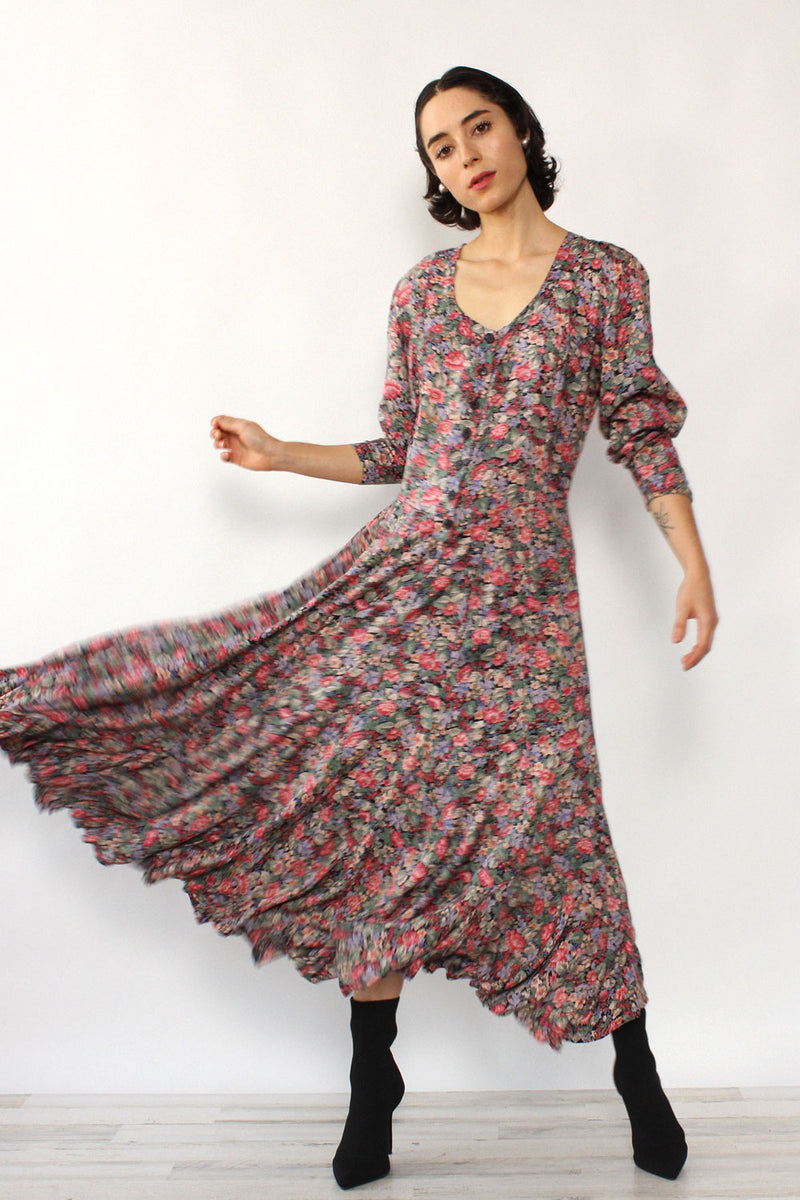In a vertical, photograph, a woman with a light tan complexion and short, dark brown hair that slightly curls at the tips stands poised and elegant. Situated just a little right of center, her head is slightly cocked to the left. Her hair ends just above her shoulders, curling gently around her neck. She wears a long-sleeved, floral dress adorned with a mix of maroon, light pink, gray, red, blue, and yellow flowers, with the sleeves rolled up just below the elbows. The dress swishes to the left, indicating movement, as if she has just spun around. Her left arm rests by her side while her right arm is bent at the elbow, extending outward. She stands on her left toe with her right foot on the ball, clad in black boots, against a light cream or white wall backdrop and a gray floor. Despite the dynamic pose and flowing dress, her expression is serious and seemingly bored, adding an intriguing contrast to the lively movement captured in the image.